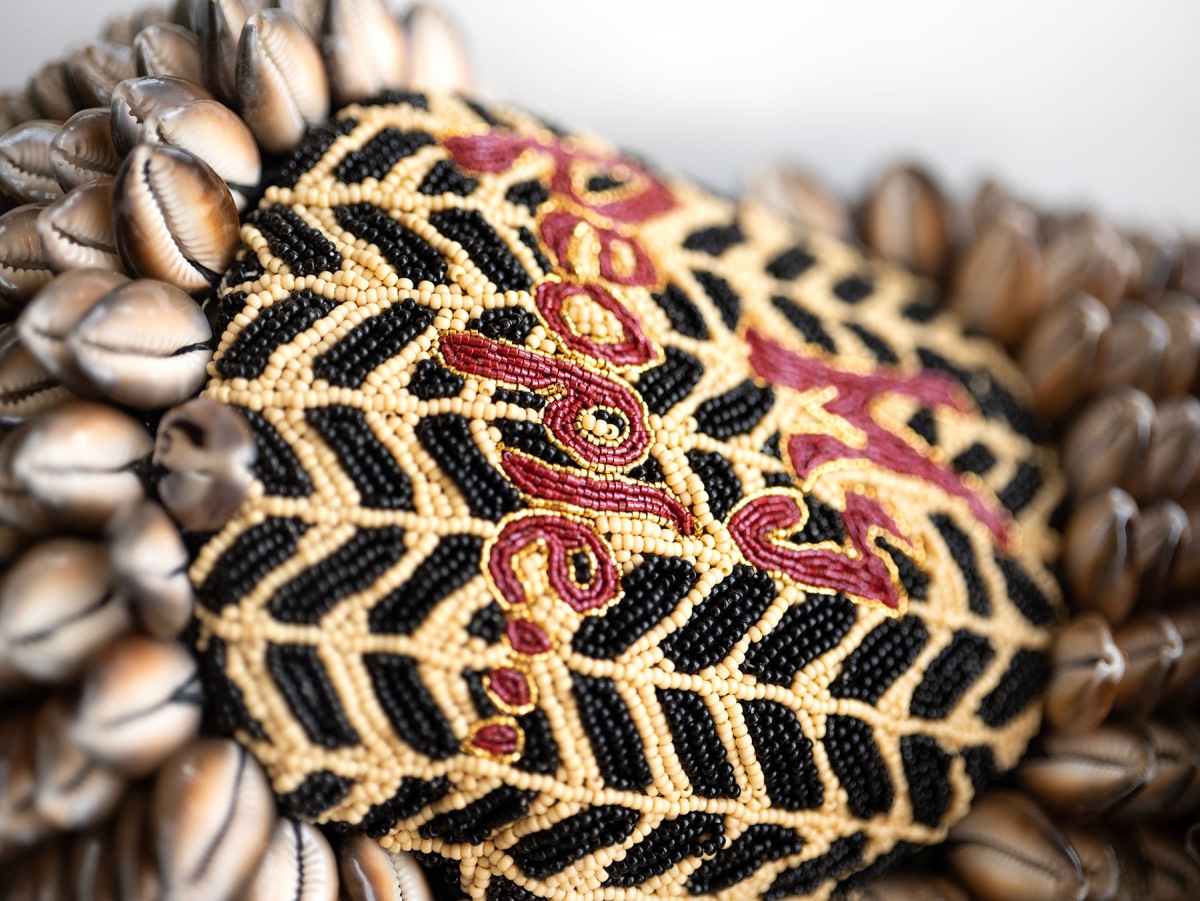The image features a unique, artisan-crafted piece that appears to be a combination of beadwork and shells, evoking the imagery of a sunflower. At the heart of the piece are intricately braided yellow and black beads, arranged in a pattern that some may liken to a zigzag or a crocheted formation. Inscribed in maroon or red and gold beads, the words "my people..." stand out prominently in the center. Surrounding this beaded core are clusters of small, tan, and brown puka shells, reminiscent of seashells found at a beach resort or tropical island. The shells create several rows, encircling the central beadwork, much like the seeds of a sunflower. The image has a slight blur, especially towards the top and the right, while the left side remains clearer, adding an enigmatic touch to this creative and culturally evocative piece.